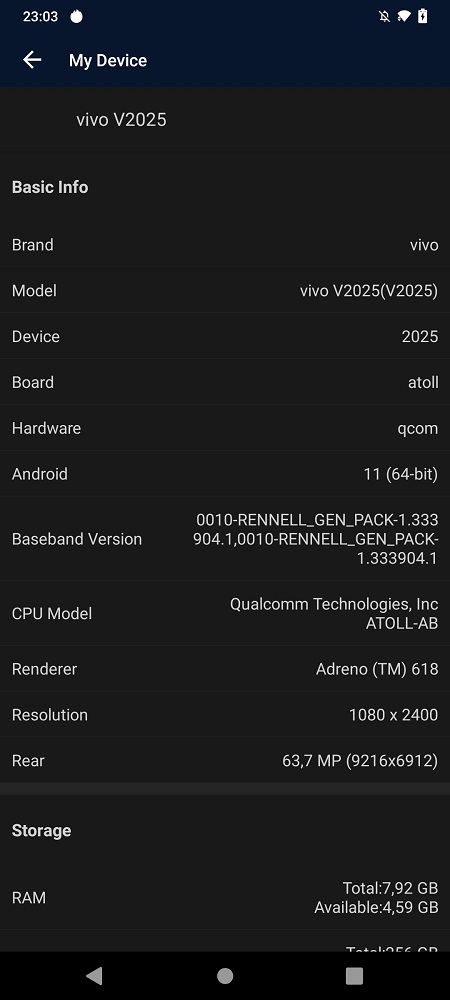This is an image of a smartphone screenshot, seemingly taken within the device's settings menu. 

**Top Section:**
- Time Display: The time is displayed in military format as "23:03."
- Status Icons: Next to the time, there's a white circle icon, a notification bell with a line through it indicating notifications are muted, and a Wi-Fi icon with an indistinguishable element to its left. The battery icon shows a full charge.

**Main Body:**
- Navigation: On the bottom left, there is a left-pointing arrow suggesting a back function, followed by the label "My Device."
- Model Information: Under "My Device," it states the phone model as "Vivo V2025" with a space separating "Vivo" and "V2025."
- Section Heading: "Basic Info" heading is below the model information.
- Device Specifications:
  - Brand: Vivo
  - Model: Vivo V2025
  - Device: V2025
  - Board: ATOLL
  - Hardware: QCOM
  - Android Version: 11, 64-bit
  - Additional Info: Contains details on CPU model, renderer, resolution, rear camera, and RAM. Notably, "Storage" is listed as a separate heading without specific details following it.

This detailed caption provides an extensive overview of the settings screen captured in the image.